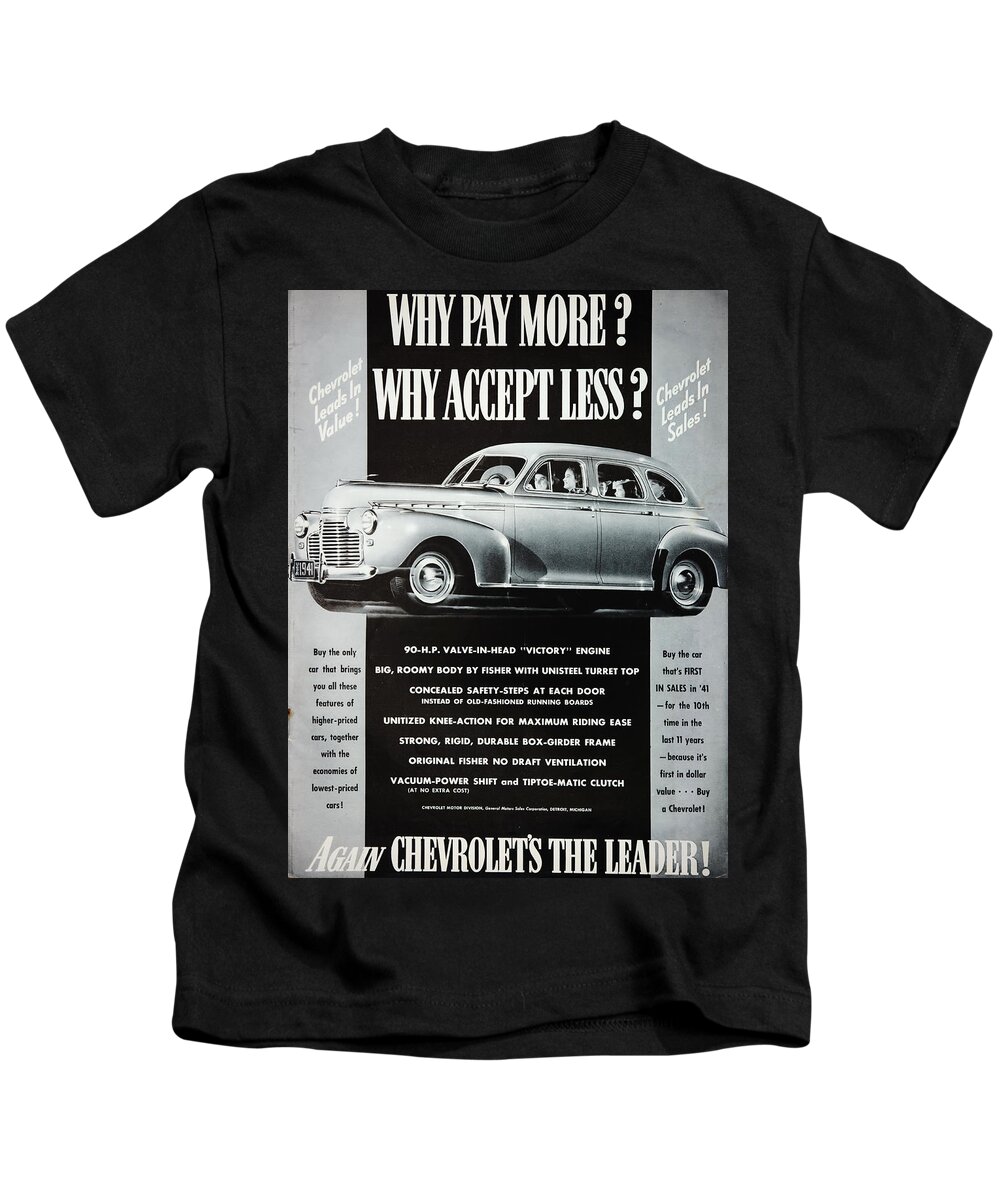This image depicts a black t-shirt with a retro automotive advertisement printed prominently on the front. Dominating the chest and stomach area, the print features a vertical design. In the center, a wide black bar runs from top to bottom, flanked by narrower light gray bars. Across the top of the black bar, bold white capitalized text reads, "WHY PAY MORE? WHY ACCEPT LESS?" Below this, an illustration of an old-fashioned, boxy vehicle with a square grille and circular headlights holds the center stage. The car is white or silver-toned, and appears to contain a family: a man driving, a woman in a sun bonnet sitting beside him, and children in the back.

Within the gray bars on either side of the vehicle, there are cursive scripts in white. On the left, the text says, "Chevrolet leads in volume," while the right side reads, "Chevrolet leads in sales." Below the car image is a line of small, illegible black text, followed by larger white text stating, "Chevrolet's the leader!" This detailed design showcases an antique Chevrolet advertisement, emphasizing the brand's leadership and value.